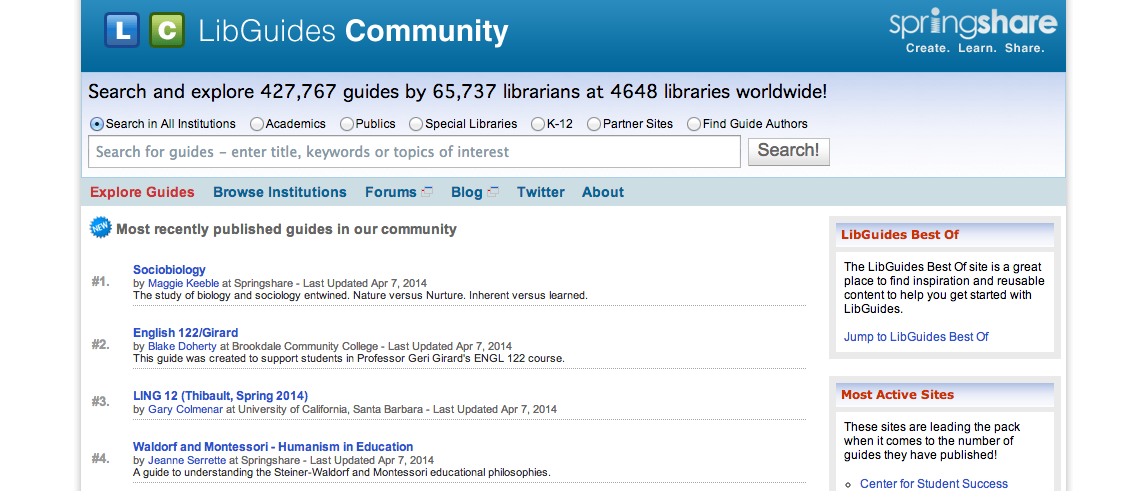**Image Description: Lib Guidelines Community Interface**

The image showcases the "Lib Guidelines Community" interface, a comprehensive platform for library resources and guides. In the upper left corner, the logo "Lib Guidelines Community" is prominently displayed. The logo comprises two boxes: a blue box with a white "L" and a green box with a white "C". Adjacent to this logo, the text "Lib Guidelines Community" is written in white font.

On the right side of the header, the platform's tagline "Spring Share: Create, Learn, Share" is displayed. Below this header, a detailed description reads: "Search and explore 427,767 guides by 65,737 librarians at 4,648 libraries worldwide."

Below this description is a set of circular icons labeled with different types of libraries and resources, including "All Institutions", "Academics", "Public", "Special Libraries", "K-12", "Partner Sites", and "Find Guide Authors". Below these icons, there is a search field labeled "Search for Guides, Enter Title, Keyword, or Topic of Interest", accompanied by a gray search button with black text.

Moving further down, there is a navigation bar with links in bold red and blue text, including "Explore Guides" (in red), and "Browse Institutions", "Forums", "Blogs", "Twitter", and "About" (in blue).

The lower section of the interface lists the "Most Recently Published Guides in our Community". The first listed guide is "Social Biology by Maggie Keeble at Spring Share", with the last update noted as "April 7, 2014". The guide delves into the study of biology and sociology, focusing on themes such as "Intertwined Nature vs. Nurture" and "Inherited vs. Learned". 

The provided description stops at the second guide, indicating there is more content following the first guide.